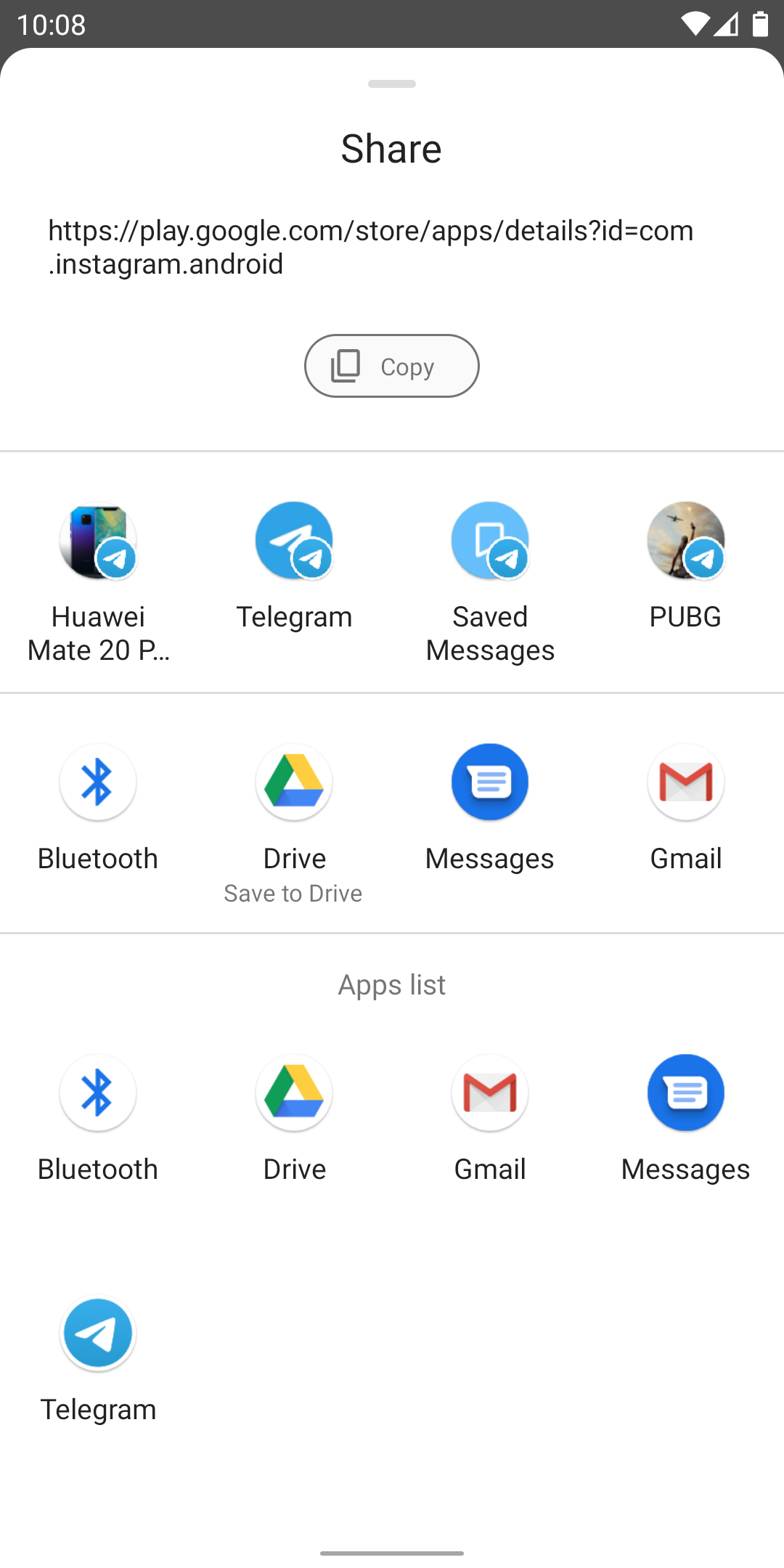This is a detailed screenshot captured from a mobile device, displaying the interface for sharing an Instagram link. The link appears to be for installing Instagram on an Android device. The sharing options are prominently displayed, featuring a large gray oval button labeled "Copy" along with 13 additional sharing options characterized by various app logos.

In the top row of sharing options, from left to right, the icons represent sharing through two different text options, "Hawaii Mate 20," Telegram, Saved Messages within Telegram, and the popular game PUBG.

The second row of options includes icons for sharing via Bluetooth, Google Drive, Messages, and Gmail.

Beneath these rows, under a section labeled "Apps list," the same four options—Bluetooth, Drive, Gmail, and Messages—are repeated. Following this, there is one more standalone option for Telegram.

In the top left corner of the phone screen, the time is displayed as 10:08. On the right side of the top of the screen, icons indicate that the battery is almost full, the device has a full Wi-Fi signal, and two out of three cellular service bars are present.